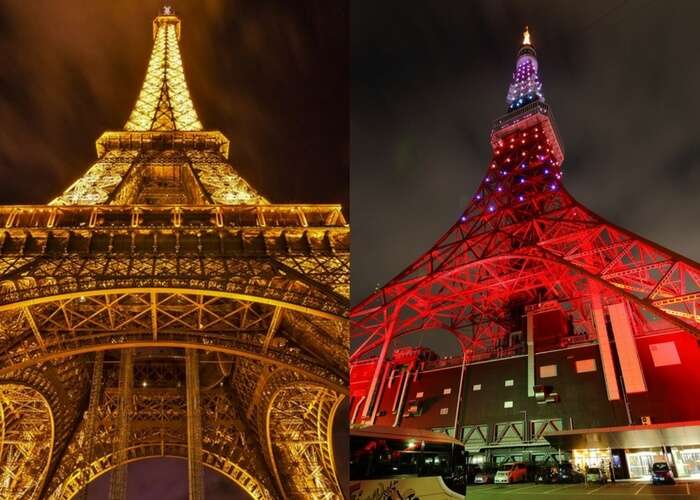The image is a side-by-side comparison of two nighttime photographs of the Eiffel Tower. In both photos, the tower is illuminated against a dark sky. The left photo presents a view from the base of the Eiffel Tower, looking up with the structure lit in golden, white-yellow lights. The angle is close and upward, capturing the full height of the tower, creating a majestic, glowing appearance. The right photo offers a more distant perspective, showing the Eiffel Tower illuminated in vibrant red and blue colors. This view allows visibility of the base of the tower, including surrounding buildings and a parking lot with vehicles. The presence of people at the bottom suggests a bustling, lively atmosphere beneath the iconic landmark.